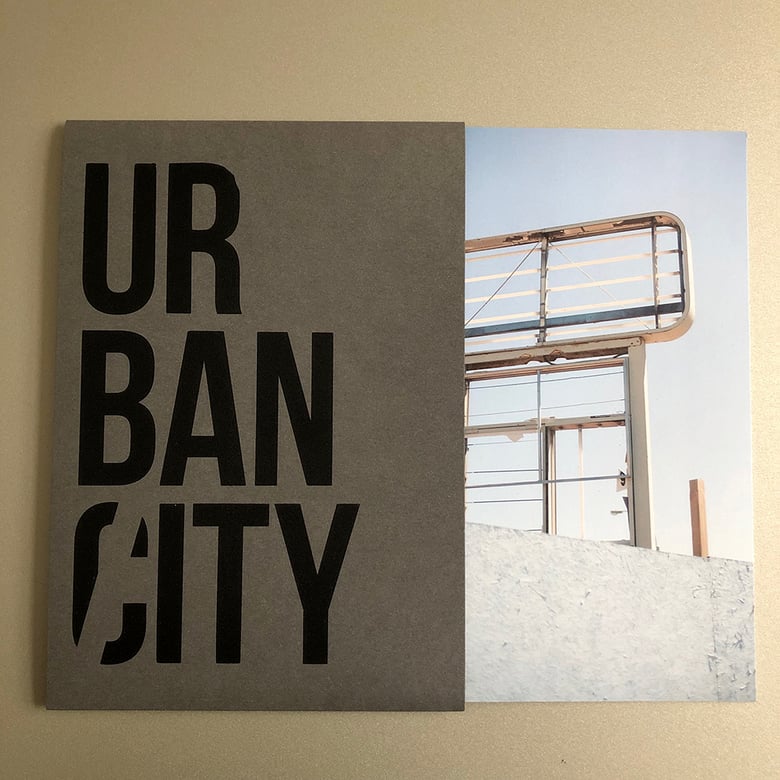This image is a detailed top view of a unique pamphlet or brochure situated on a white desktop. The left side of the pamphlet is slightly larger than the right, and when opened, the right side's image will be fully revealed. The solid light brown background frames the pamphlet, centering it perfectly. The left side features a dark brown, textured cover resembling cardboard or fabric. Large black letters printed in all caps spell out "URBAN CITY" over three lines. The text has a high-contrast design with the letters 'C' in 'CITY' featuring a distinct strike-through. On the right side, there's an intriguing photograph displaying urban decay: a cement wall with a skeletal signpost emerging from it, devoid of any signage, surrounded by clear blue sky and some visible wires. The combination of these images strongly suggests the pamphlet addresses issues related to urban maintenance, abandonment, and decay.